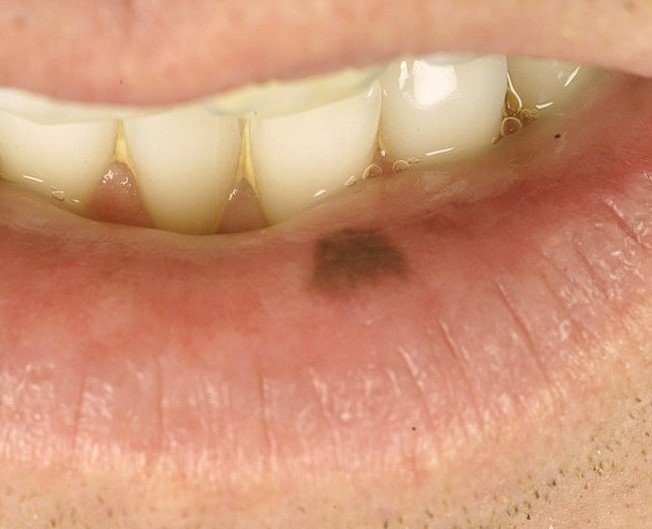This is an extreme close-up photograph of a person's partially open mouth, revealing their lips and teeth. The lips, primarily pink and moist, feature a distinctly noticeable square patch of dark pigmentation on the lower lip, potentially indicative of a medical condition or skin abnormality. The top lip is minimal, appearing mostly as skin, while the bottom lip has some visible dark stubble suggesting the person is likely a man. Near the stubble on the bottom lip, there's a freckle or small dark spot. The teeth, mostly white, are somewhat compromised by yellow plaque, particularly between the two front teeth, and there is visible saliva inside the mouth expressed as small bubbles. The intricate details of the lips show natural wrinkles and a light brownish area, emphasizing the possible significance of the pigmentation. The image lacks any background, focusing entirely on the mouth area, making it clear and detailed for examination purposes.